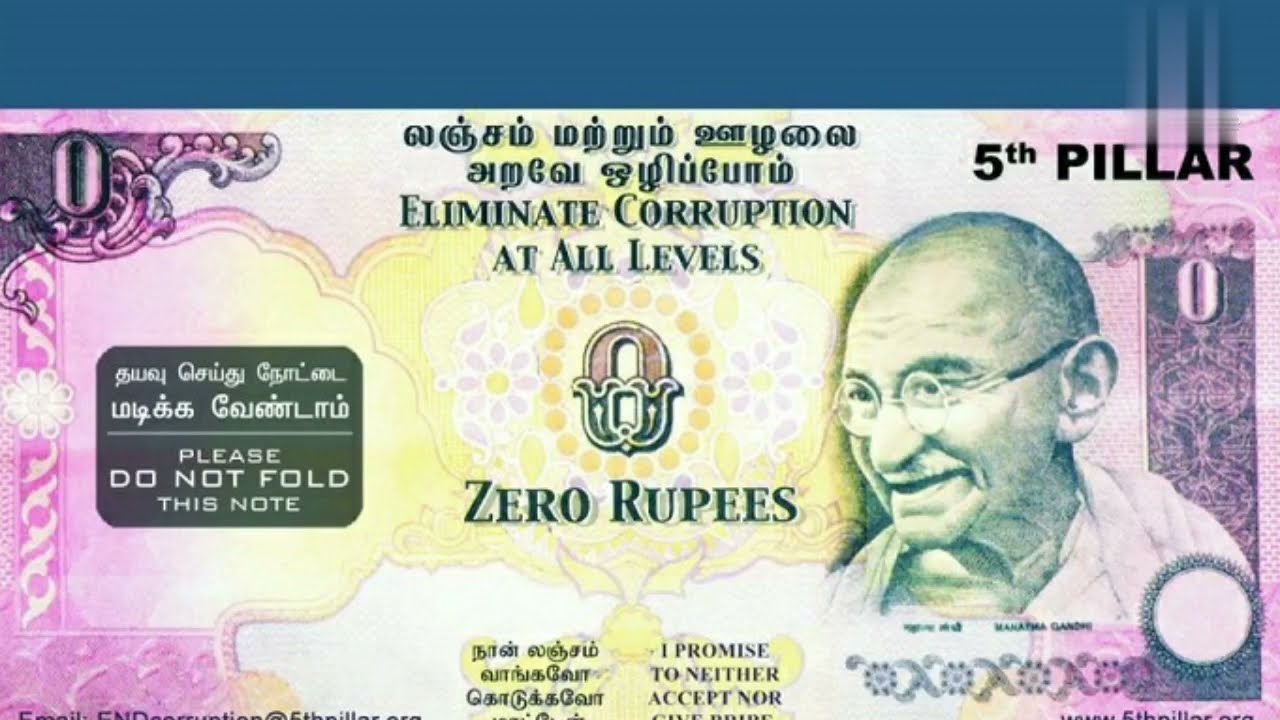This image depicts a large and elaborately designed note resembling a rupee, set against a dark blue background. The primary design of the note features a bright purple coloration with a prominent yellow hue in the center. Inscribed in the upper left-hand corner is the number zero, which is repeated in the middle of the note beneath an intricate design. The central part of the note also bears the phrase "Eliminate corruption at all levels" in black text. The upper right-hand corner reads "Fifth Pillar," possibly indicative of the issuing organization or a movement. Below the phrase "zero rupees," there is a partially visible text declaring, "I promise to neither accept nor," suggesting an anti-corruption message. The left side of the note features a gray box with the instruction, "please do not fold this note," written in English. On the right side, there is a smiling portrait of Mahatma Gandhi, identifiable by his glasses. Surrounding this image are various elements that further enhance the note's appearance as a piece of currency, although it clearly functions symbolically to promote a stance against corruption.